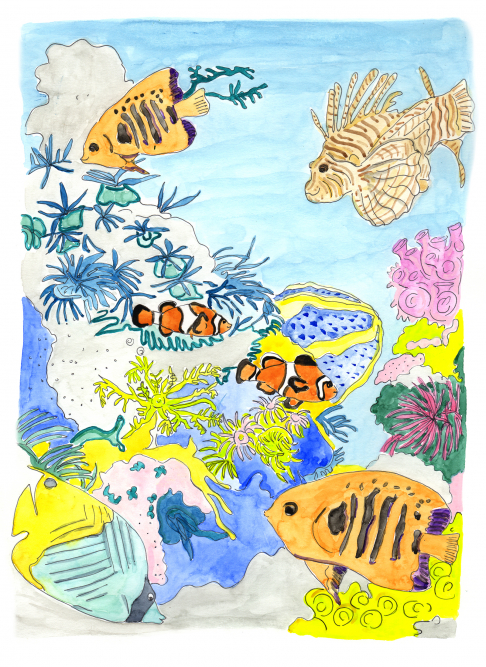This detailed drawing, created with felt markers, vividly depicts an underwater scene, possibly in a fish tank or the ocean. At the center, two iconic clownfish, with their distinctive orange, white, and black stripes, are prominently featured. Above them, a vibrant orange fish and a majestic lionfish with its characteristic fins and stripes swim gracefully. Below the clownfish, a yellow-tailed, blue-bodied fish, and another fish with an orange body adorned with a hint of purple can be seen. The background showcases a mesmerizing light blue expanse of water, punctuated with mounds of sand and sea plants. The scene is enriched with diverse coral formations in hues of whites, blues, yellows, and purples, and a pink coral nestled to the right. The upper right corner of the drawing features an impressive lionfish, while other animated fish populate the reef. Open water lies at the top, adding to the depth and tranquility of this rich aquatic tableau.